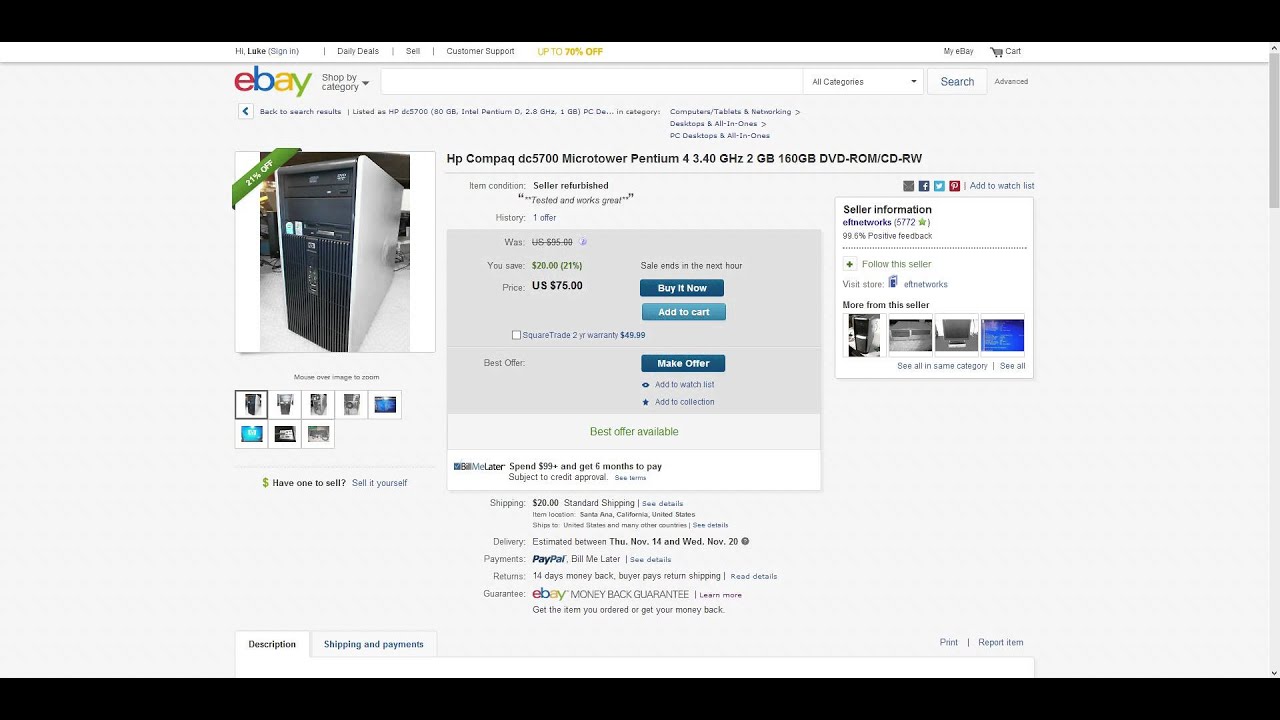This is a detailed image of a web page from eBay. The top and bottom of the screen feature black borders, while the main section of the page is a very light gray. At the top, eBay's header includes five small, unreadable tabs and a shopping cart icon on the right.

Below the header, the word "eBay" is prominently displayed next to "Shop by Category." An adjacent search box includes a drop-down menu to select "All Categories" and a search button.

The central photo is of an HP Compaq DC5700 Micro Tower. The tower has a sleek design, with a black front and a white body. The listing details it as having a 4.3 GHz Platinum processor, 2 GB of RAM, and a 1600 GB hard drive. It includes a DVD-ROM and CD-RW drive. Additionally, there are eight supplementary photographs of the product.

The item is listed for $75, with options to "Buy It Now," "Add to Cart," or "Make Offer." Social media icons below the listing allow sharing on Facebook, Twitter, Pinterest, and another unidentified platform.

A section for seller information is present but too small to read clearly, displaying four thumbnail images. Following this are more unreadable text sections. 

At the bottom, there are visible tabs for "Shipping and Payments" and "Description," with an option to "Report" on the right.